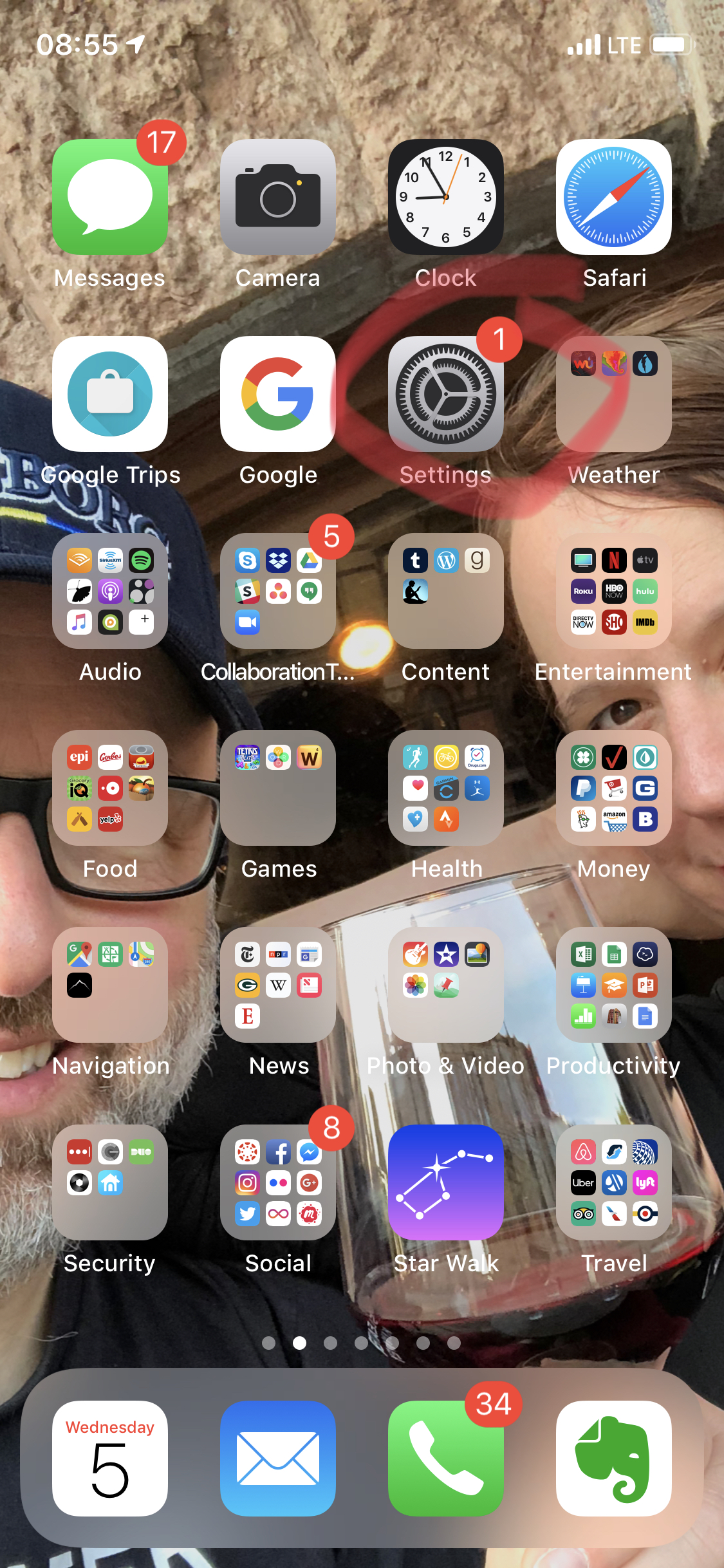This image showcases the screen of an iPhone with a detailed display of various elements on it. At the top left corner, the time is indicated as 8:55 AM with a small white arrow adjacent to it. The top right corner features the signal strength bars, "LTE" icon, and a battery indicator that appears nearly full.

The phone's wallpaper is a photograph of a man and a partially visible woman. The man, positioned on the left, is wearing a dark blue baseball cap displaying the letters "B-O-R-G" and a pair of black-rimmed glasses. He has a short beard and mustache; his beard is mostly gray while the mustache is a darker shade. He is dressed in a black shirt. The woman on the right side of the image is leaning on her right arm, but most of her face is cut off from the frame. She has brown hair. Between them stands a glass of red wine that is almost empty, though enough remains to identify it as red wine.

On the phone screen, several app icons are displayed, many of them indicating unread notifications. The text messages app shows a red bubble with the number 17, the settings icon displays a red bubble with the number 1, a folder labeled "Collaboration" has a red bubble with the number 5, another folder labeled "Social" displays a red bubble with the number 8, and the phone app shows a red bubble with the number 34.

Additional app icons visible on the screen include Camera, Clock, Safari, Google Trips, Google Weather, Audio, Content, Entertainment, Food, Games, Health, Money, Navigation, News, Photo and Video, Productivity, Security, Star Walk, and Travel.